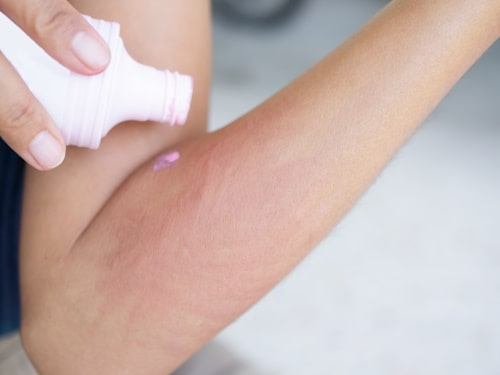The photograph captures a woman's arm, prominently displayed against a white background. Her arm is bent at the elbow with the elbow situated at the bottom left of the image and the wrist area extending toward the top right, positioning the forearm diagonally across the photo. She is applying a pink ointment, likely calamine lotion, to a reddish, bumpy abrasion near the bend of her elbow. The ointment is dispensed from a small white bottle, held by her short-nailed fingers, which are positioned at the top left of the image. Only her arm and the bottle are visible, with the lotion forming a distinct dot on the irritated skin.